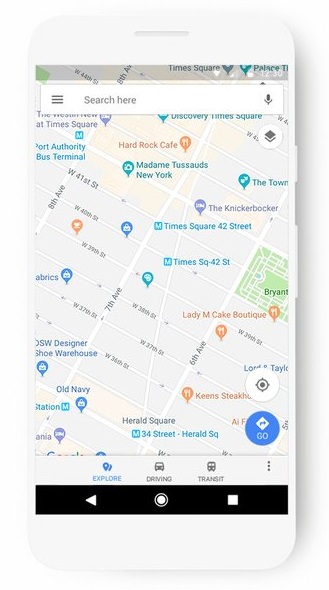The image showcases an older model iPhone displaying a zoomed-in map of a city, likely New York City. Prominent landmarks such as Hard Rock Cafe, Times Square, Herald Square, and The Knickerbocker are clearly labeled, suggesting the map is centered around a bustling area of Manhattan. At the top of the screen, a search bar is visible, allowing users to enter terms to search for different locations. At the bottom, there is an interactive "driving" button, presumably for obtaining driving directions to the highlighted area.